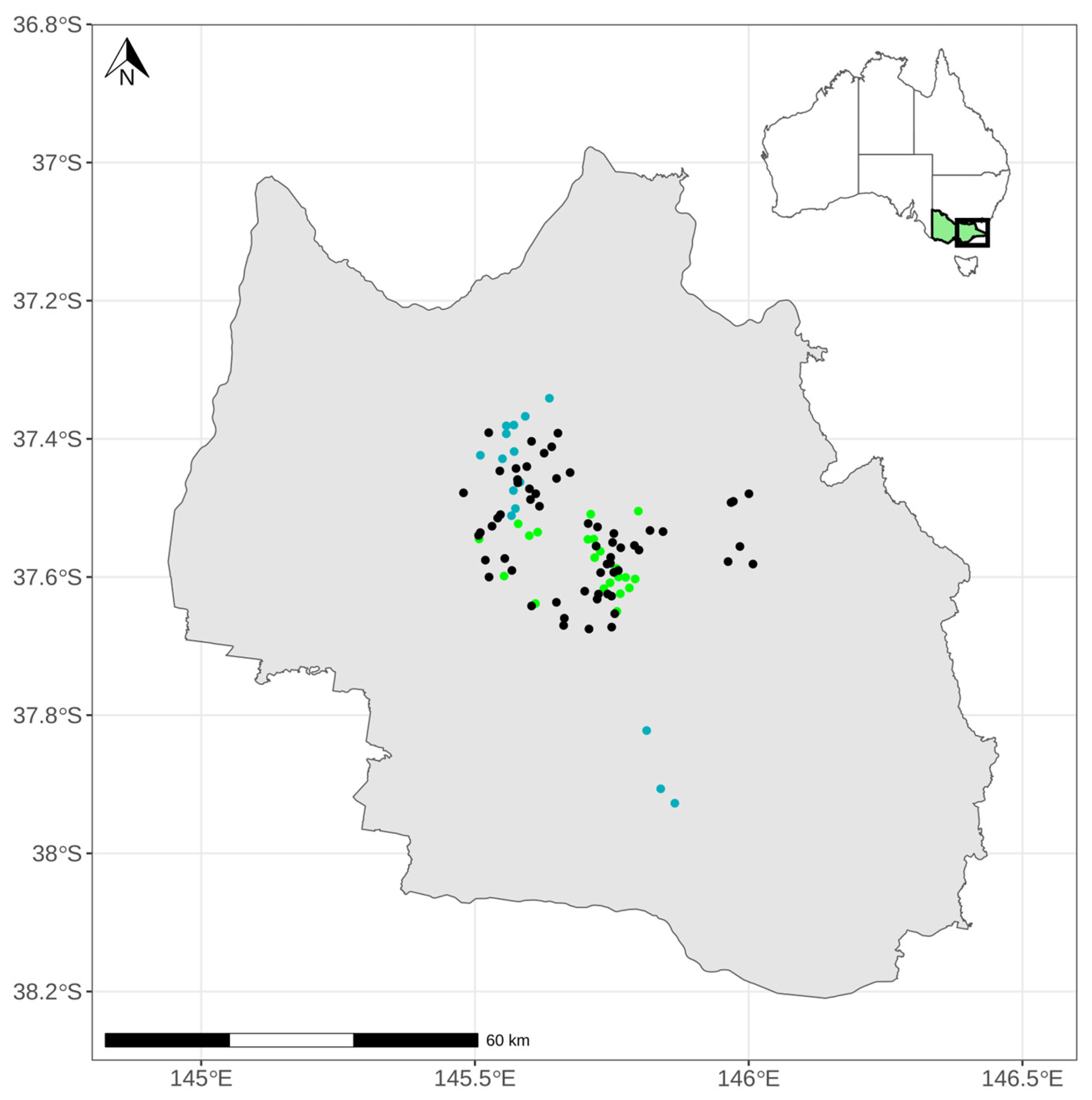This image features a detailed map focusing on a specific section of southeastern Australia, prominently marked and highlighted for emphasis. In the top right corner, an outline of the entire Australian continent is shown with a black square pinpointing the area of interest. The main section of the map, displayed in gray, covers latitudes from 38.2°S to 36.8°S and longitudes from 145°E to 146.5°E. The area within the black square, in the lower right-hand portion of Australia, is colored in green, providing visual contrast.

Clusters of dots in various colors—black, blue, and neon green—are largely concentrated in the center of this detailed region. Smaller groups of blue dots are scattered towards the bottom, while some black dots are situated off to the right. The entire map is overlaid with a grid, and the coordinates along the axes are clearly labeled: the Y-axis on the left side reads from 38.2°S at the bottom to 36.8°S at the top, and the X-axis at the bottom spans from 145°E to 146.5°E. This setup, complete with numbers and lines, underscores the precision and specificity of the geographic focus.